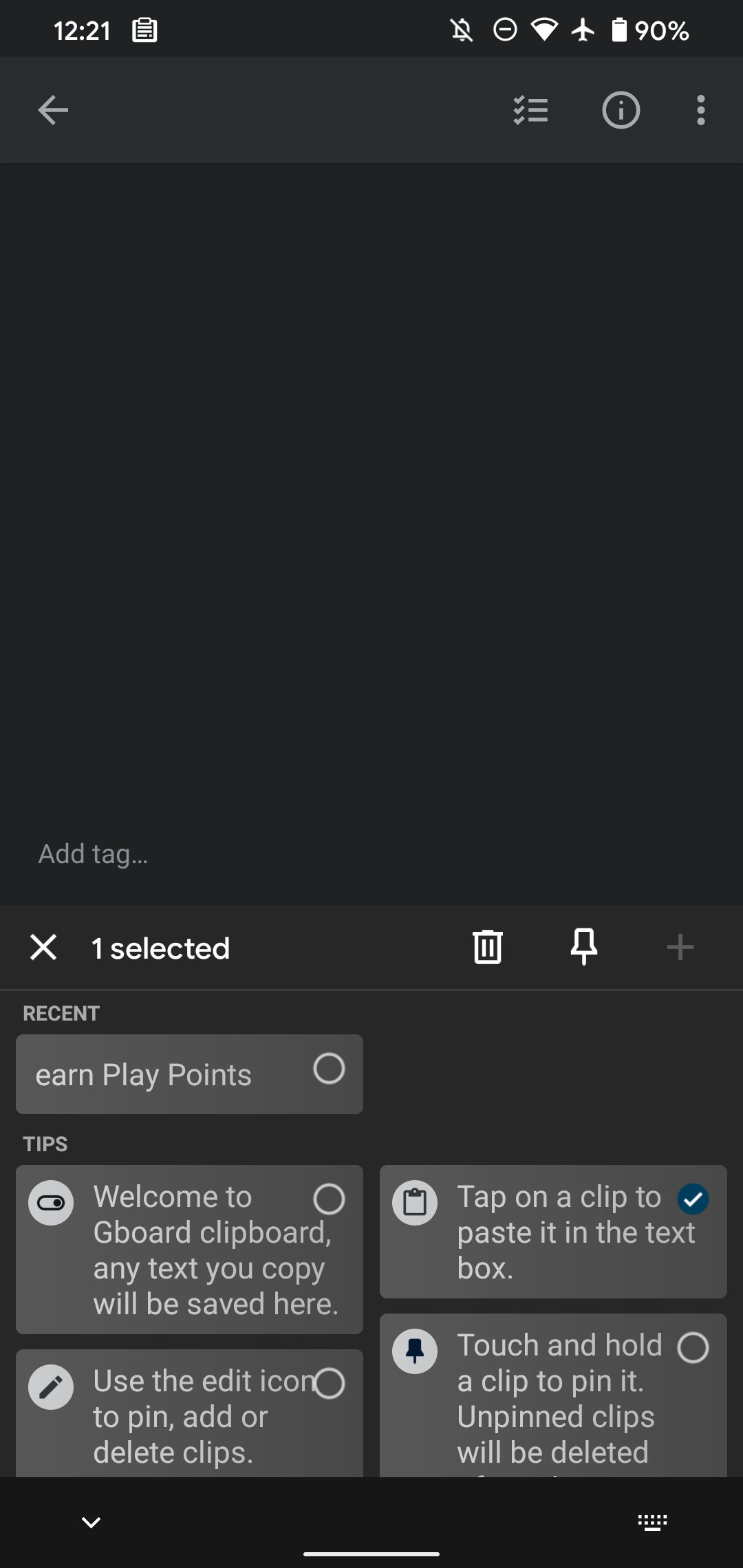The image depicts a smartphone screen displaying a digital interface, primarily the clipboard function of a keyboard app, likely Gboard. At the top of the screen, the status bar shows the current time as 12:21, along with various icons including an airplane mode symbol, battery percentage, and a muted notification bell, all rendered in white on a black background. Below the status bar is a search field with additional icons, such as an eye within a circle and a three-dot menu, suggesting options for adjusting settings or accessing more functionalities.

Underneath the search field, the interface presents a section titled "Add tag," indicating one tag is selected, accompanied by icons for deletion (trash bin), cancellation (X), and pinning (pin), all in white. Below this section, within the "Recent" label, there’s an option titled "Earn Play Points" with a selectable circle, followed by a "Tips" section. 

The "Tips" detail the functionality of the clipboard:
1. A welcome message to Gboard Clipboard, explaining that any text copied will be saved there, and instructing users to tap on a clip to paste it in the text box. This section features a pencil icon.
2. A note on using the edit icon to pin, add, or delete clips, alongside a pin icon.
3. Instructions on touching and holding a clip to pin it, mentioning that unpinned clips will be deleted.

The majority of the screen features a sleek design with a black background and white text, contributing to a minimalist and user-friendly interface.